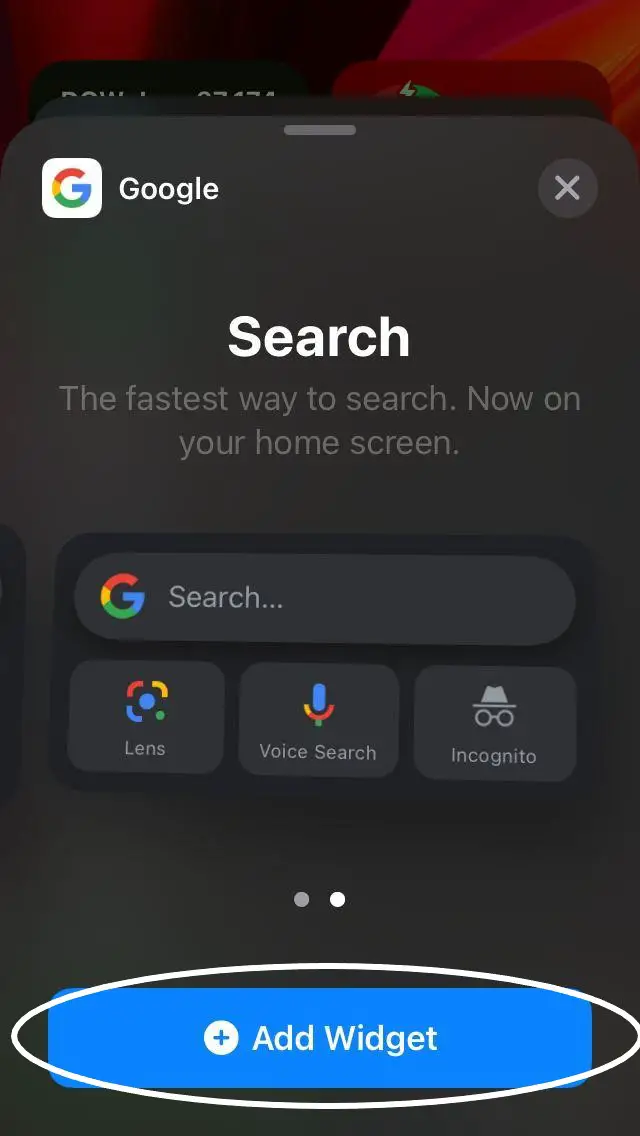The image features a smartphone screen showcasing a menu overlay in the foreground. The backdrop of the screen displays a red and black gradient, visible at the very top. Dominating the foreground is a dark gray menu that has been pulled up from the bottom. In the top left corner of this menu is a prominent white "G" logo, followed by the word "Google" written in white text to its right. On the opposite top right corner, there's a small gray circular icon with an X inside it.

Directly beneath this header, centered on the screen, is a message stating, "Search, the fastest way to search now on your home screen," accompanied by the Google search bar below it. Following the search bar are four icons arranged in a grid: Google Lens, Voice Search, and Incognito mode. Below these icons, two small white dots indicate the menu's pagination.

At the very bottom of the screen, a blue button stands out. This button features a white circle with a blue plus sign in the middle and is labeled "Add Widget" to the right of the plus sign. The "Add Widget" label is emphasized by a surrounding white oval. Additionally, at the top of the screen, you can spot a small white square with the recognizable colorful Google "G" logo.